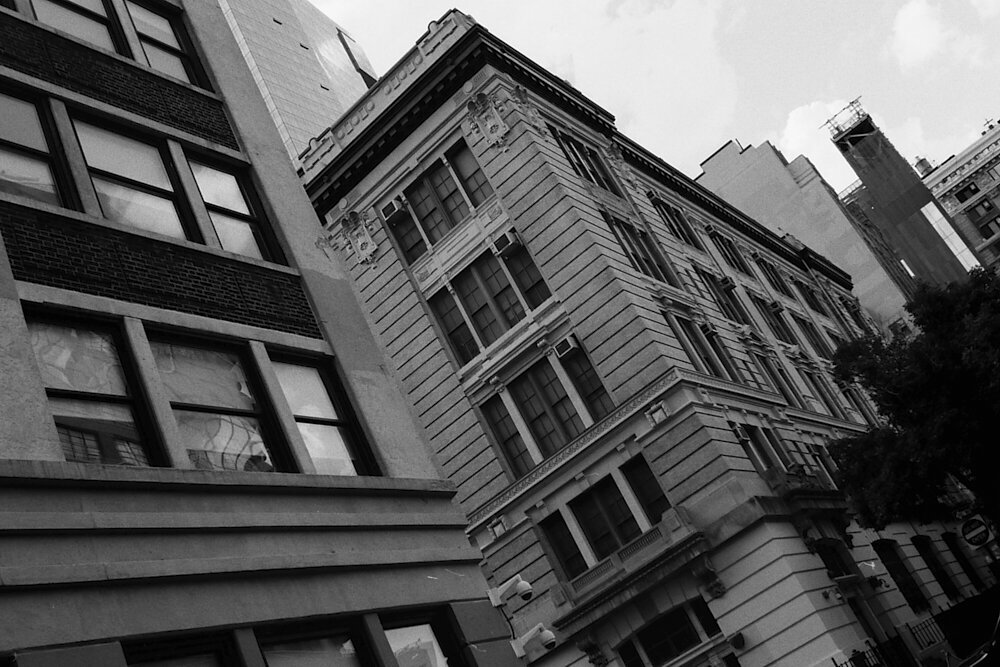This striking black-and-white photograph artfully captures a cityscape, where various buildings, seemingly tilting to the left due to the photographer's skewed angle, create a sense of dynamic tension. The foreground is dominated by an older, turn-of-the-century building with four to five stories, showcasing stonework and horizontal siding. In front of this structure and partially visible, the image reveals another building featuring darker exposed brickwork. A tree stands on the sidewalk in front of these buildings, adding a touch of nature to the urban scene. Behind them rises a more modern, multi-story building constructed from concrete, brick, and glass. The background's tall skyscrapers, with their shiny metal and glass facades reflecting the sunlight, contrast strikingly with the older architecture. Light, fluffy clouds adorn the sky, further enhancing the photograph's depth and complexity. Notably, a "Do Not Enter" one-way street sign and modern security cameras on the nearest building confirm the photograph's contemporary setting, despite its vintage, grayscale appearance.